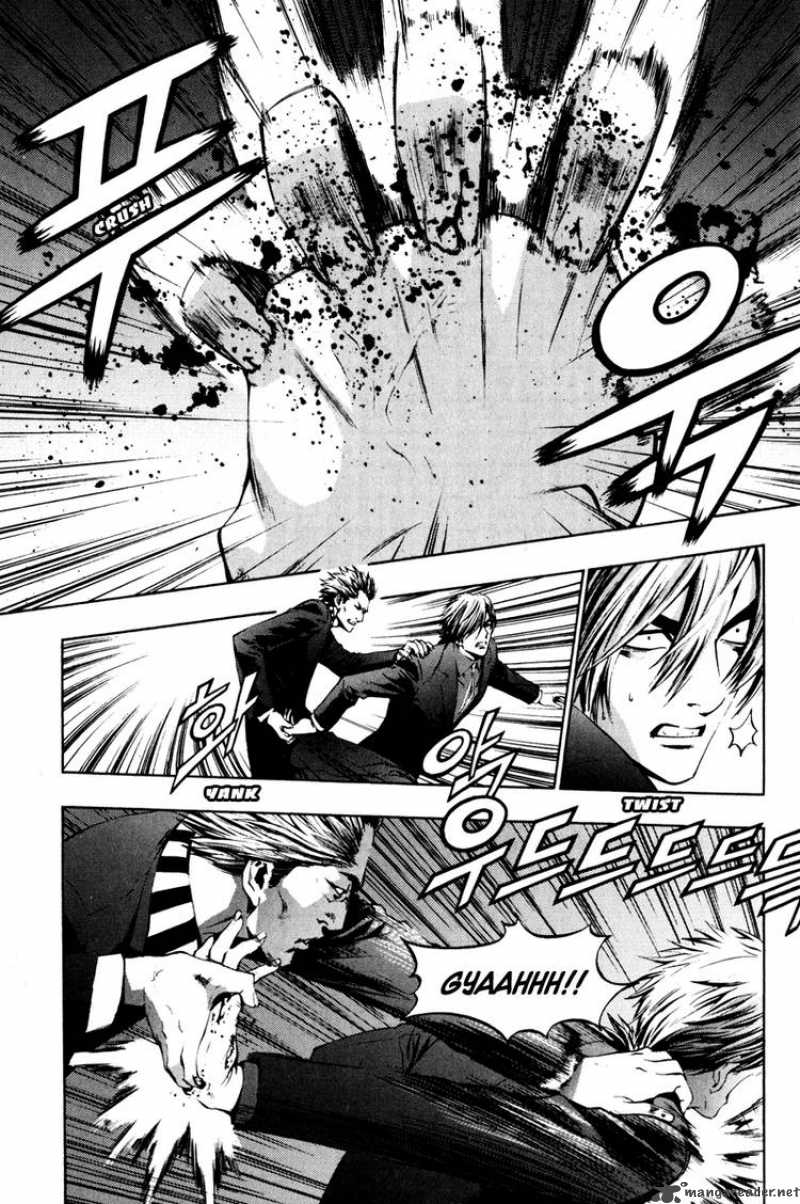This image is a detailed black and white page from a comic book, divided into three distinct frames, each packed with action and emotion. The top frame, the largest of the three, depicts a dramatic close-up of a hand with fingers curled into a claw-like position, surrounded by what appears to be spattered blood, emphasizing a violent impact. Embedded in this scene is text, both in English and Korean, with the English word "Crush" and the Korean onomatopoeia "Poo-ook" conveying the sound of the forceful action.

The middle frame continues the intense action, showing a man grabbing another from behind with significant force, further depicted by the Korean word "Hwa-ak" and the English phrase "Yank and Twist." A close-up of the aggressor’s face reveals a look of intense determination or anger, while the victim exhibits clear distress. This frame suggests a struggle, with the aggressor dominating the scene.

In the bottom frame, the conflict reaches a climax as the dominant man twists the other's arm, possibly breaking it, while pushing him down. The text shows the victim's anguished scream "Kya!" and a string of Korean characters "Oo-duh-duh-duh-duh-duh-duh-duh-duh-duh," adding to the auditory assault of the scene. Both men are depicted in detailed attire, reinforcing the dramatic intensity of this black-and-white comic book page.